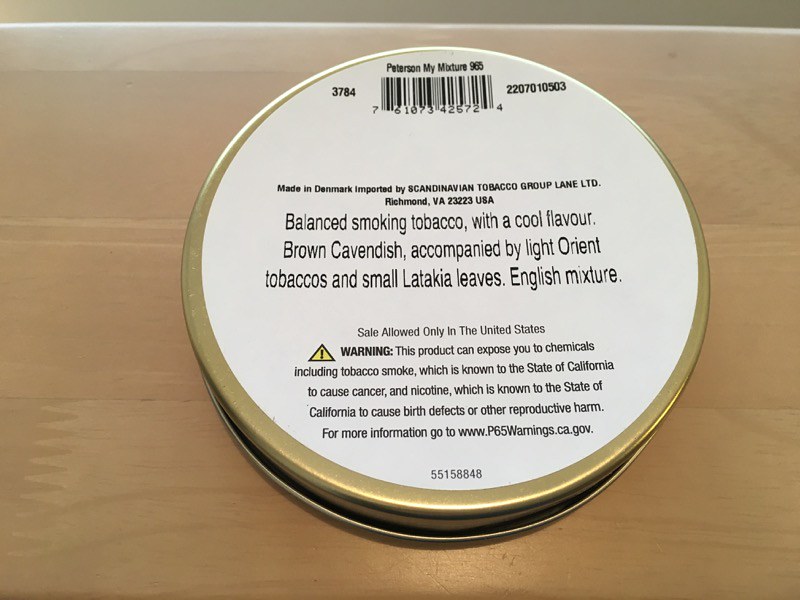The image depicts the underside of a tobacco tin, flipped upside down. The canister features a gold rim and a white and black label. At the top, it reads "Peterson My Mixture 965." The barcode at the top displays the numbers 61073 425724. Additional numerical codes on the left and right sides state "3784" and "2207010503" respectively. The label specifies that the product is made in Denmark, imported by the Scandinavian Tobacco Group, Lane LTD, Richmond, VA 23223, USA. The main text in black highlights, "Balanced Smoking Tobacco with a cool flavor, Brown Cavendish, accompanied by light orient tobaccos and small latakia leaves, English mixture." Below, it indicates "Sale allowed only in the United States." A health warning mentions that the product contains chemicals known to cause cancer and birth defects, directing users to visit p65warnings.ca.gov for more information.